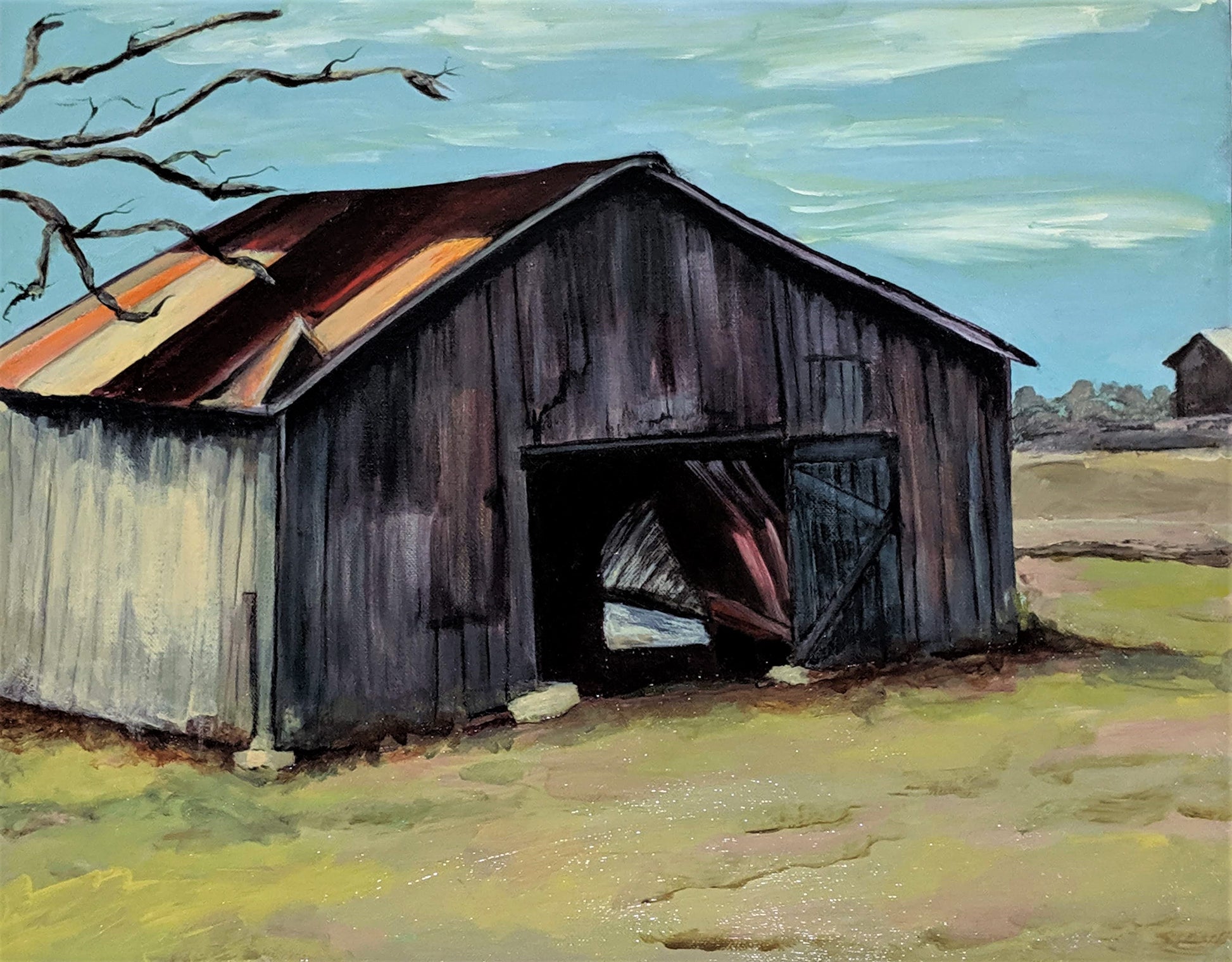This rectangular oil painting, approximately six inches wide and four to five inches high, presents a detailed landscape featuring an old, dilapidated barn set against a vast field and sky. The bottom half of the painting showcases a field rendered in tones of yellowish-green and grayish-green, with patches of pinkish-brown dirt visible in the lower right-hand corner. The upper half captures a blue sky streaked with long, thin horizontal clouds that transition from white in the center to gray and green at the edges.

Dominating the painting is a weathered barn made of gray vertical wood, accented with bits of red. The barn, which occupies the center-left of the composition, features an open doorway revealing a dark interior. The structure appears to be precariously supported by what seems to be chunks of cement. Its roof, depicting various degrees of rust, combines tones of black, grayish-white, and orange and is partially bent, suggesting significant disrepair.

In the upper left corner, a few bare branches of a tree protrude into the scene. In the background on the right side, a smaller barn or shed is just visible, providing depth to the composition. This secondary structure is accompanied by tiny trees, enhancing the desolate yet realistic atmosphere of the painting. The meticulous details and nuanced colors effectively convey a sense of abandonment and decay, capturing the essence of a neglected rural landscape.